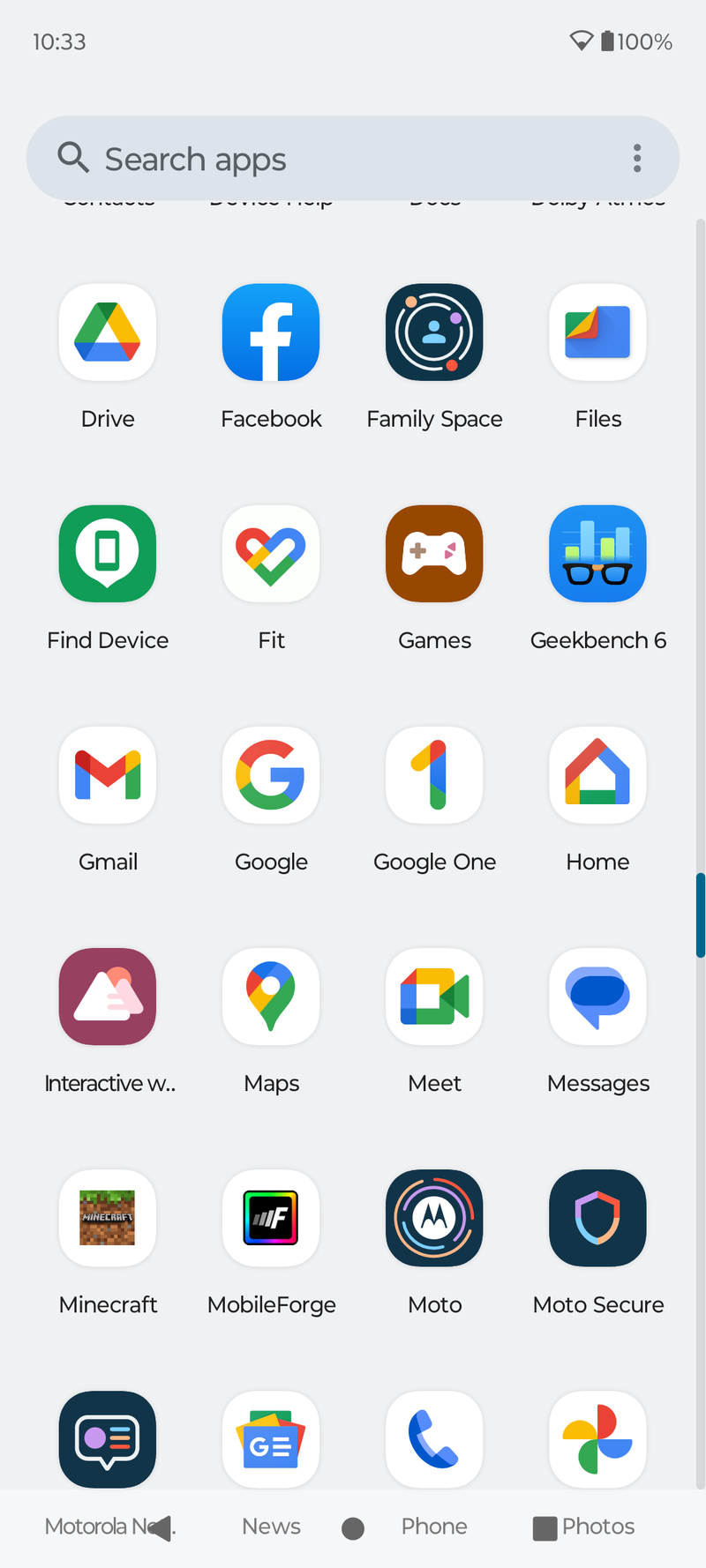This screenshot showcases the application search interface on an Android phone, identifiable by the presence of Google applications and the familiar Android design. At the top, the status bar displays the time at 10:33 in the top left, with Wi-Fi signal strength and a fully charged battery icon in the top right. Just below, a search bar is positioned, featuring a magnifying glass icon and the prompt "Search apps," flanked by three horizontal dots on the far right.

Below the search bar, the screen lists various installed apps in a grid format. The apps are arranged from left to right in the following sequence: Drive, Facebook, FamilySpace, Files, Find Device, Fit, Games, Geekbench 6, Gmail, Google, Google One, Home, Interactive W, Maps, Meet, Messages, Minecraft, Mobile Forge, Moto, and Moto Secure. The final row includes Motorola (partially obscured by a navigation button), News, Phone, and Photos.

At the very bottom of the screen, a navigation bar consists of three buttons: back, home, and a square-shaped button whose function is not immediately clear. The back button partially covers the name of the Motorola app, making it difficult to decipher the complete name. The overall background of the interface is an off-white color, providing a neutral backdrop for the app icons and text.